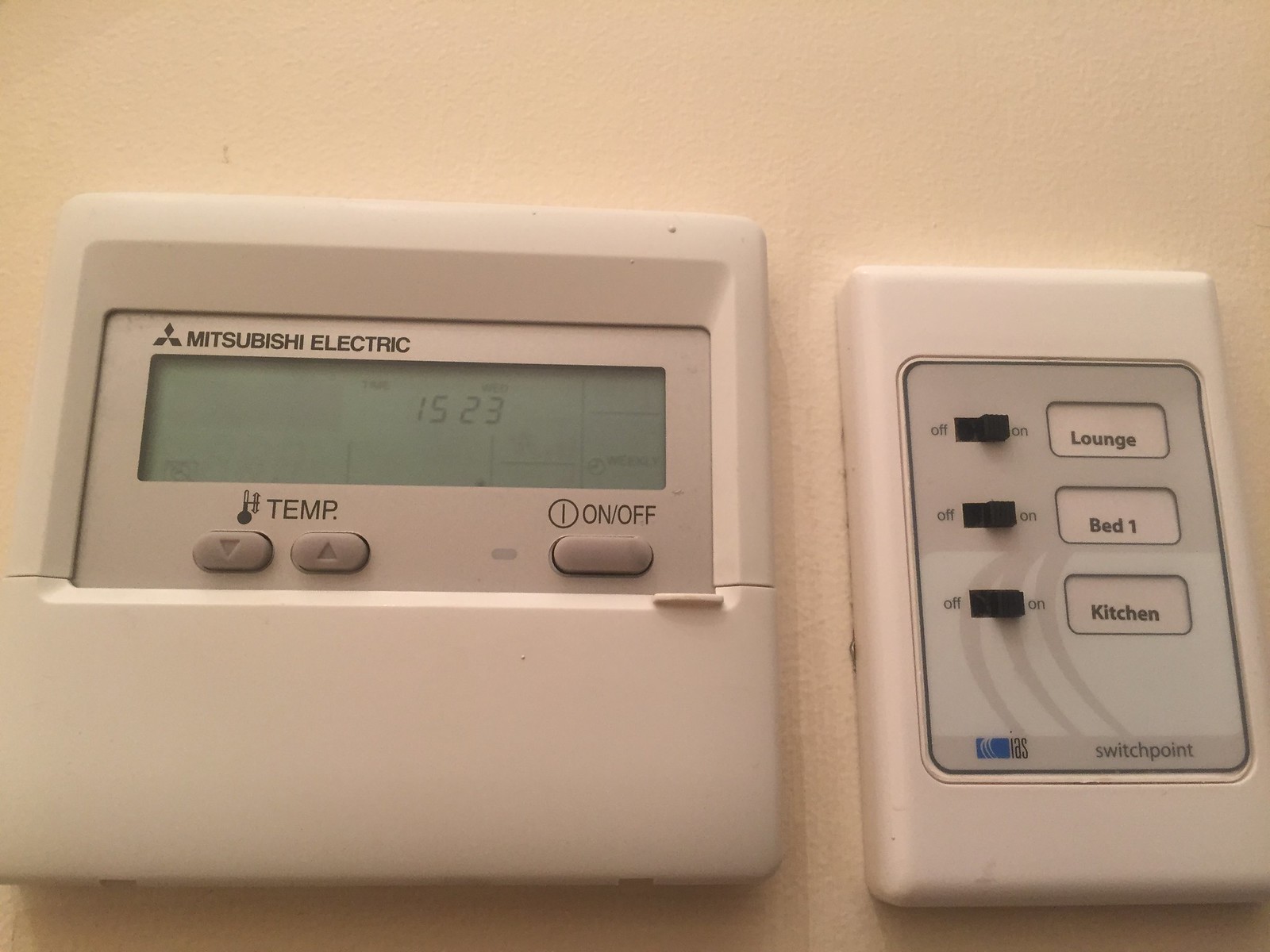This image captures two electronic devices mounted on a light pinkish-orange wall. On the left, a digital thermostat encased in white plastic prominently features a digital display showing the number '1523'. Below the display are two buttons marked with upward and downward arrows, and the label "TEMP" is printed in black above them, next to what appears to be a bulb. To the right of the display is an oval button labeled with "ON/OFF" alongside a small circle with a vertical line inside. The words "Mitsubishi Electric" are written above the display, accompanied by the Mitsubishi symbol of three black diamond shapes on the left.

On the right side of the wall-mounted setup is another device framed in either white or beige plastic, equipped with three black switches arranged vertically. Each switch is labeled "ON" and "OFF" and is adjacent to a small rectangular label indicating the area it controls. The top switch label reads "LOUNGE," the middle switch label reads "BED 1," and the bottom switch label reads "KITCHEN." Below these switches, the word "SWITCHPOINT" is inscribed in black letters. To the left of "SWITCHPOINT," there is a blue symbol containing white curved lines with the acronym "IAS" printed in black.